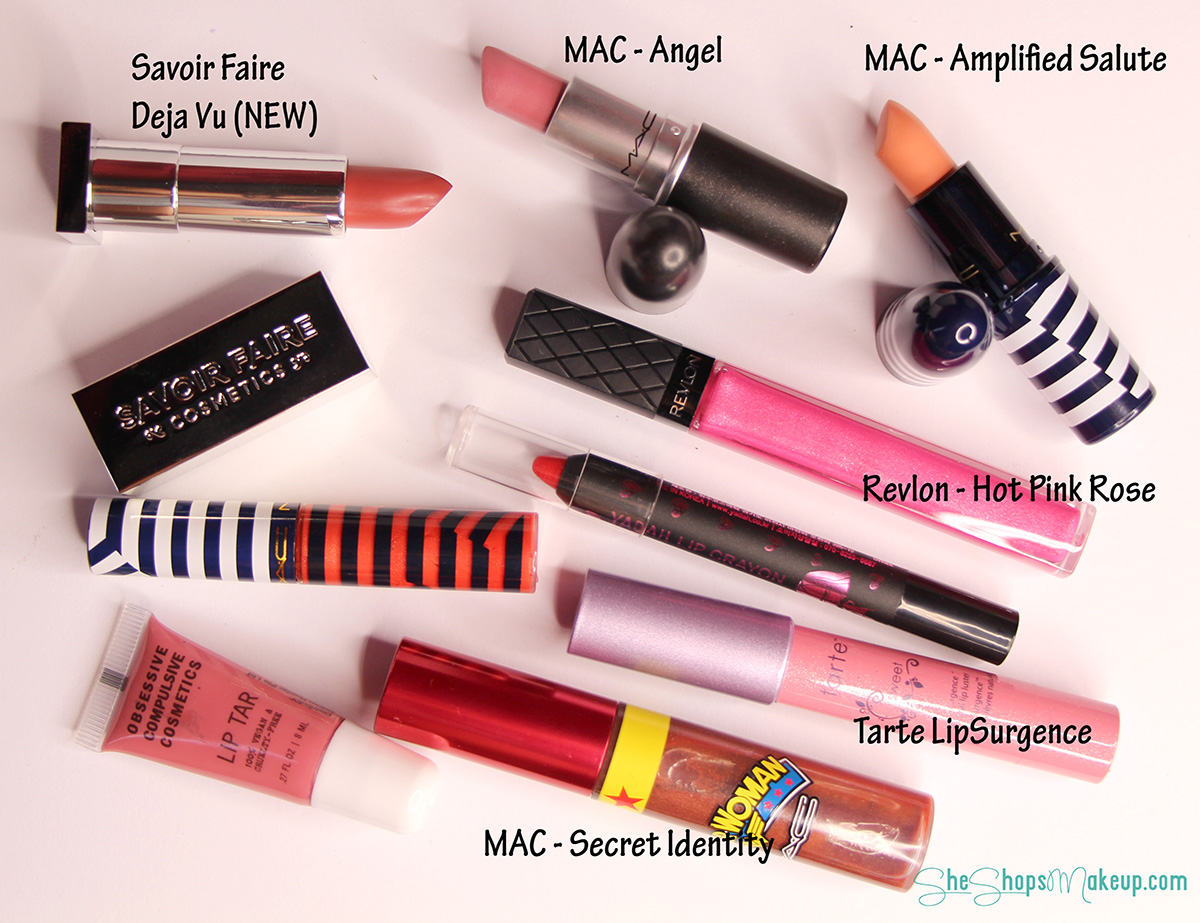The image features an array of various makeup items related to lip care and enhancement, meticulously arranged on a light pink background. There are different types of lipsticks and lip-related products, including lip tars in plastic tubes. Some lipsticks have been exposed to reveal their shades, adding vibrant colors to the scene. The items are labeled with annotated text in black, detailing brand names and product titles such as "Severe Fear Deja Vu," "Mac Angel," "Mac Amplified Salute," "Revlon Hot Pink Rose," "Tarte Lip Surgeons," and "Mac Secret Identity." Additionally, a label in the bottom right corner in blue text reads "She Shops Makeup.com." The photograph is taken from an overhead perspective, showcasing the makeup items with a cohesive pink hue emanating from both the products and the background surface.